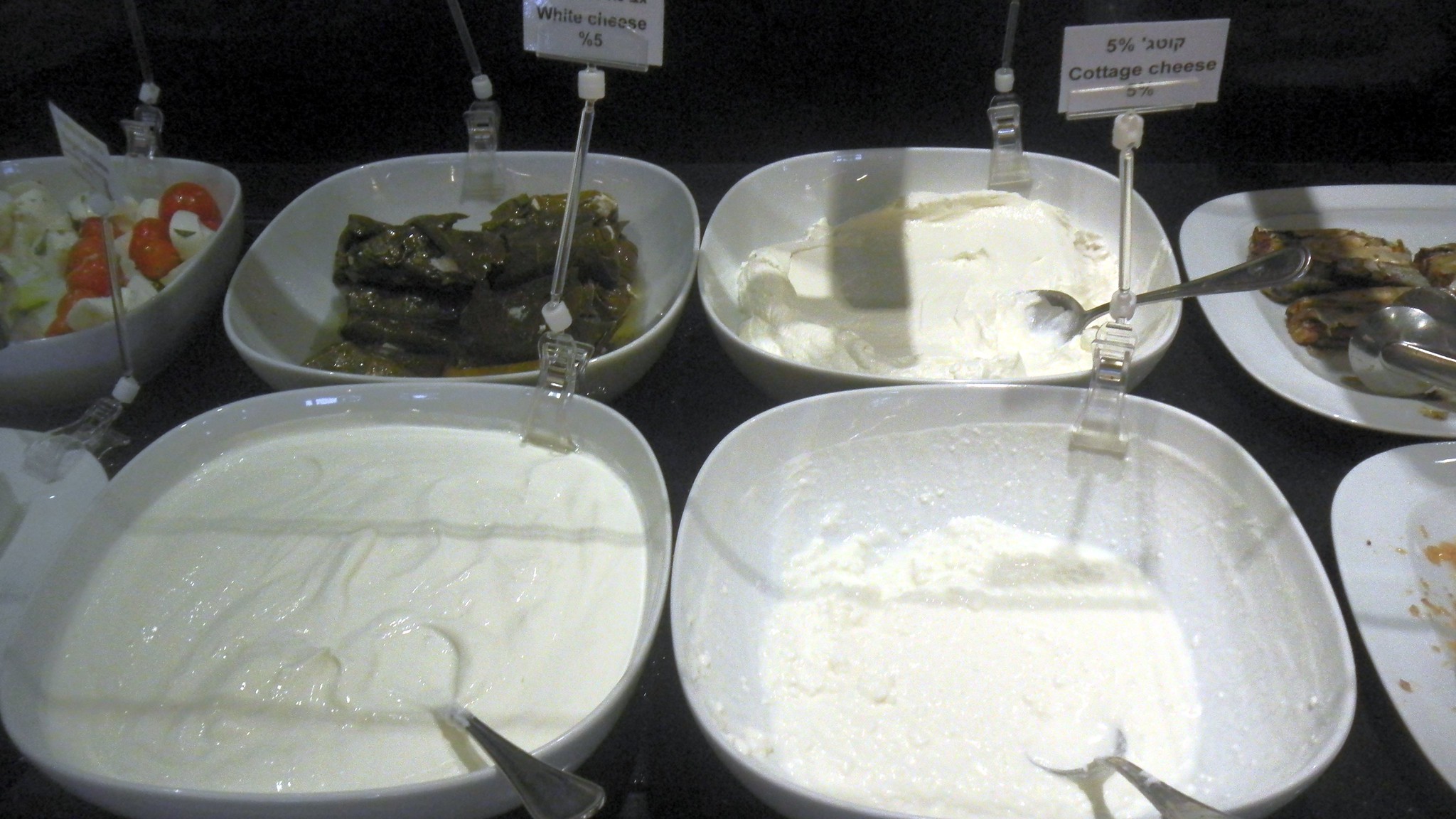This image depicts a buffet-style deli counter with an array of white bowls neatly lined up, each containing distinct food items. Prominently in the foreground are two bowls labeled "cottage cheese" and "white cheese," both equipped with metal serving spoons. The cottage cheese bowl's spoon appears well-used, while the white cheese bowl’s spoon looks unused. Behind these, there is a selection of salad ingredients including green vegetables like possibly cooked green beans and small tomatoes. Towards the back, there's a bowl filled with what appear to be pickled jalapeños. The display also includes a plate with a portion of meat accompanied by serving tongs. Visible signage marked "5%" indicates some form of percentage notation for the dishes. The overall scene is set against a dark background, enhancing the focus on the vividly white dishes and their diverse contents.